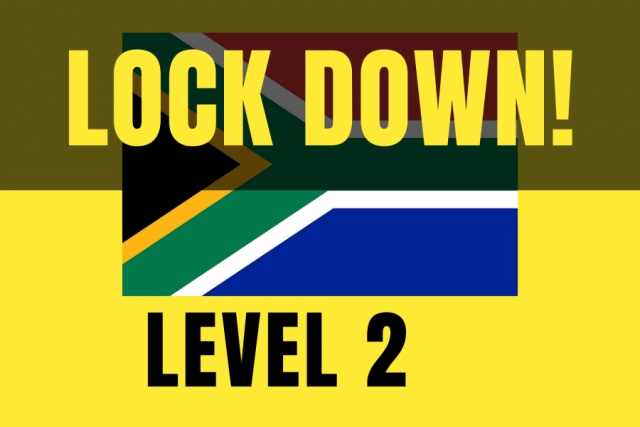The image depicts a public announcement sign for "Lockdown Level 2." The background is divided into two distinct colors: the bottom half is solid yellow, while the top half is a military green or dark gray-yellow. Centered on the image is a flag featuring a variety of colors including red, blue, black, yellow, green, and white. The flag has a Y-shaped design with its fork towards the left and a straight down section to the right. The Y is green, surrounded by lightly colored gray stripes, with a yellow V inside and areas of black, red, and blue. At the top of the image, the word "Lockdown!" is prominently displayed in light yellow text, superimposed over the military green background. The bottom half of the sign contains the text "Level 2" in black, set against the yellow background. The overall style suggests an informational poster alerting viewers to the lockdown status.